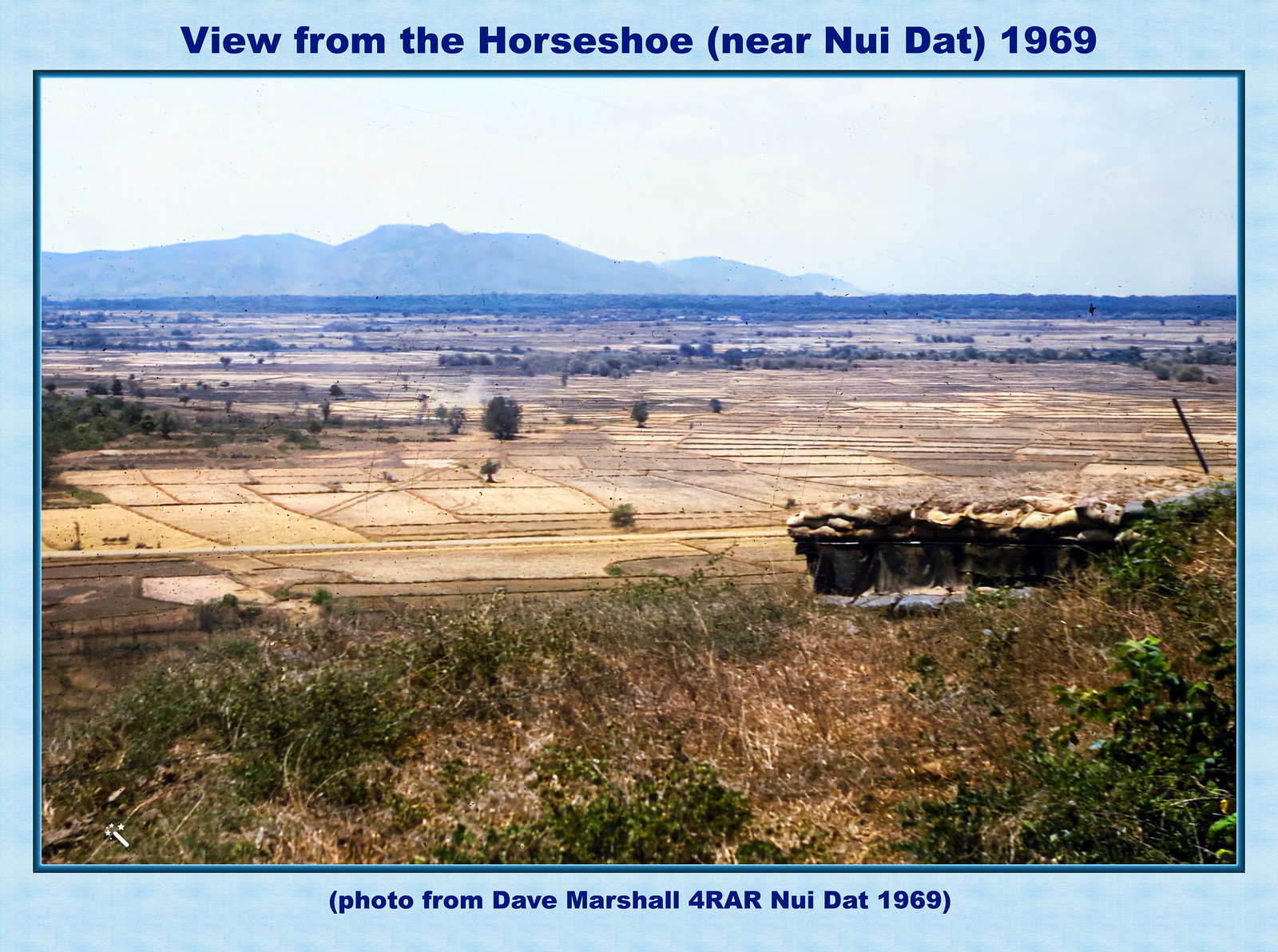This landscape photograph, bordered with a light blue frame and dark blue captioning, is titled "View from Horseshoe near Nui Dat, 1969" and was taken by Dave Marshall for RAR (Royal Australian Regiment). The image, likely from Vietnam during the Vietnam War era, depicts a scene from an elevated vantage point, possibly a hill. The foreground features scrubland with brownish grass, green weeds, and a few black buckets, potentially filled with rocks. Moving further back, there are sparse sandbags suggesting bunkers, indicative of military presence. The middle ground consists of wide, open plains with dirt and sand, occasionally dotted with bushes, resembling sown fields or paddies. In the hazy background, the terrain transitions to distant hills or mountains under a clear, light blue sky with occasional clouds. Despite the age and slight washout of the photograph, the scene vividly captures the sparse, yet strategic, landscape near Nui Dat in 1969.